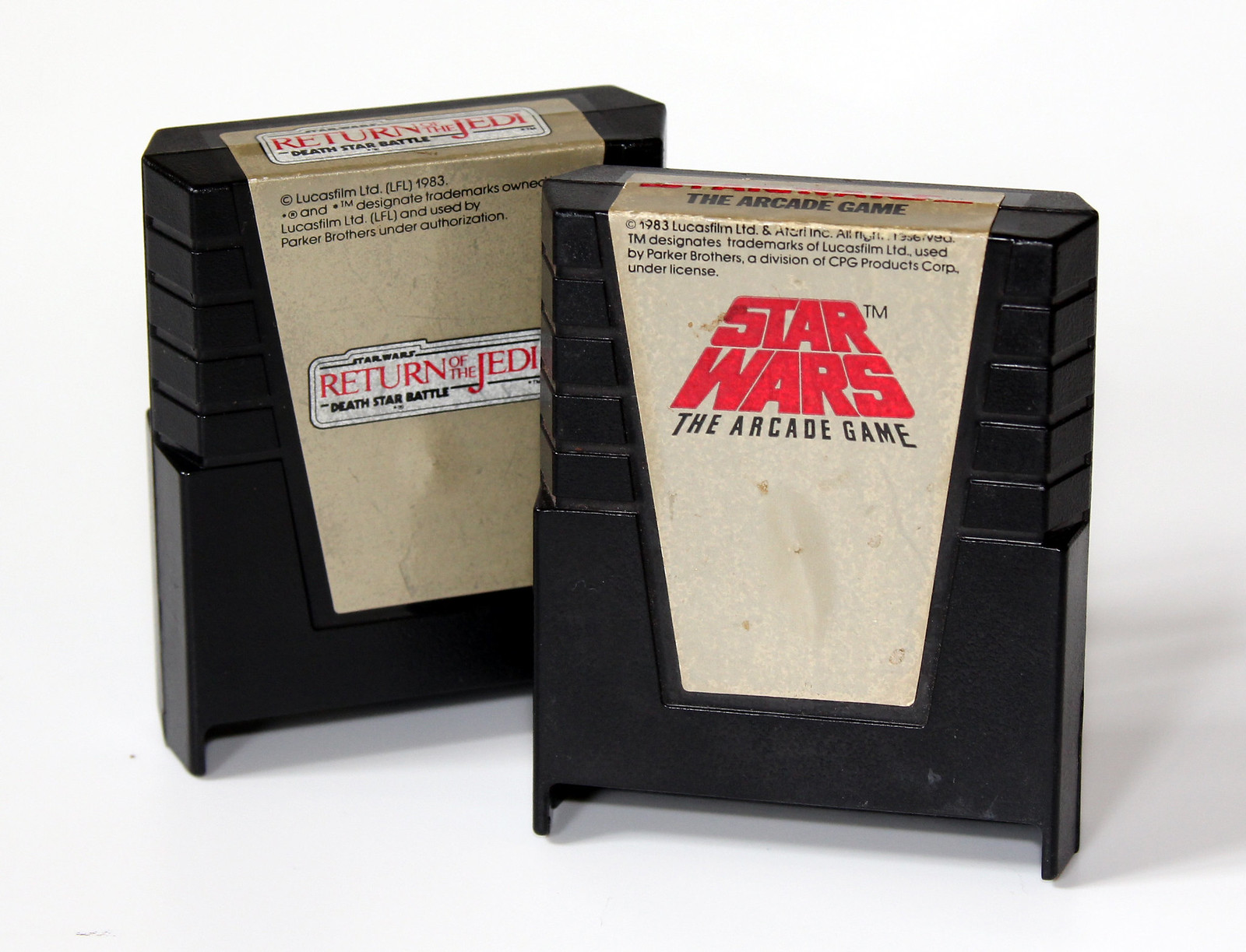In this professional photograph, two vintage black gaming cartridges stand upright against a stark white background. The cartridge on the left features a white label that reads "Star Wars: Return of the Jedi - Death Star Battle," along with the year "1983" and trademark information like "Lucasfilm Ltd." and "used by Parker Brothers under authorization." The cartridge on the right is labeled "Star Wars: The Arcade Game," also from "1983," featuring similar trademark details but noting its license under "CPG Products Corp." Both cartridges, reminiscent of classic Atari games, showcase their titles prominently and include various regulatory and credit text, collectively evoking a nostalgia for early '80s arcade gaming.